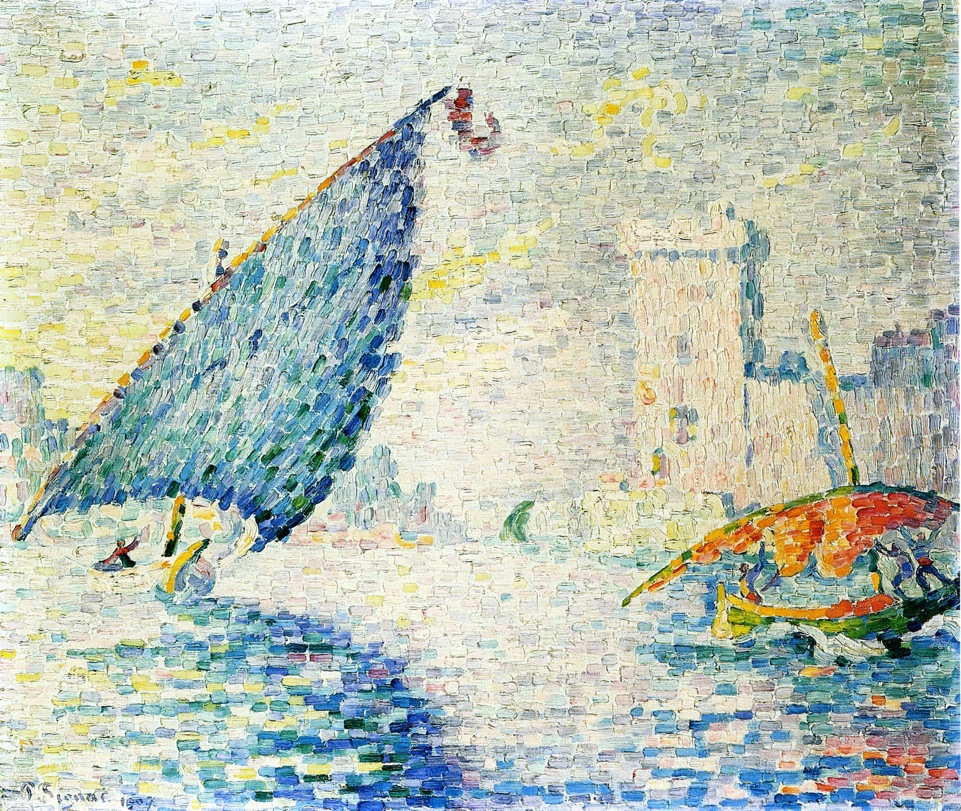This is an abstract square painting featuring a seascape with multiple boats and buildings in the background. The sky is depicted with hues of yellow, white, and light blue, while the water is a blend of blue, green, yellow, and white. In the lower right of the image, there is a boat with its sail down, alongside three people working around it. To the lower left is a small sailboat with a solitary figure, who is wearing a red shirt. The sailboats show vibrant colors—the sails include shades of blue, green, yellow, red, and orange. In the background, there are buildings, which appear large and ancient, with some resembling Venice Canal structures. These buildings are painted with white and have a brick-like texture due to the short, horizontal brushstrokes. The overall scene is impressionistic, with detailed strokes creating a sense of motion and light, highlighting the serene yet bustling activity on the water.